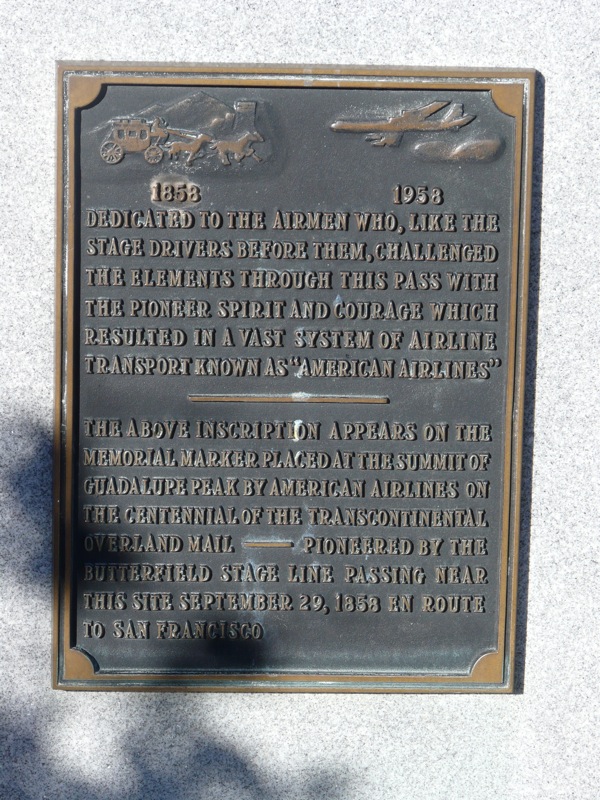This image captures a bronze engraved plaque mounted on a light-colored gray and white stone or marble wall at the summit of Guadalupe Peak. The plaque, bordered in gold with raised gold letters, is dedicated to the adventurous airmen who, like the stage drivers before them, braved the elements through the pass with pioneer spirit and courage. These efforts contributed to the development of the extensive airline transport system known today as American Airlines. On the upper left of the plaque, there is an engraving of a horse-drawn stagecoach marked with the year 1858, while the upper right features an engraving of an airplane marked with the year 1958. This plaque was placed by American Airlines to commemorate the centennial of the transcontinental overland mail service pioneered by the Butterfield stage line, which passed near this site on September 20, 1858, en route to San Francisco. The photograph also shows a shadow from a nearby tree or bush in the bottom left corner, further enhancing the outdoor setting of this historical marker.